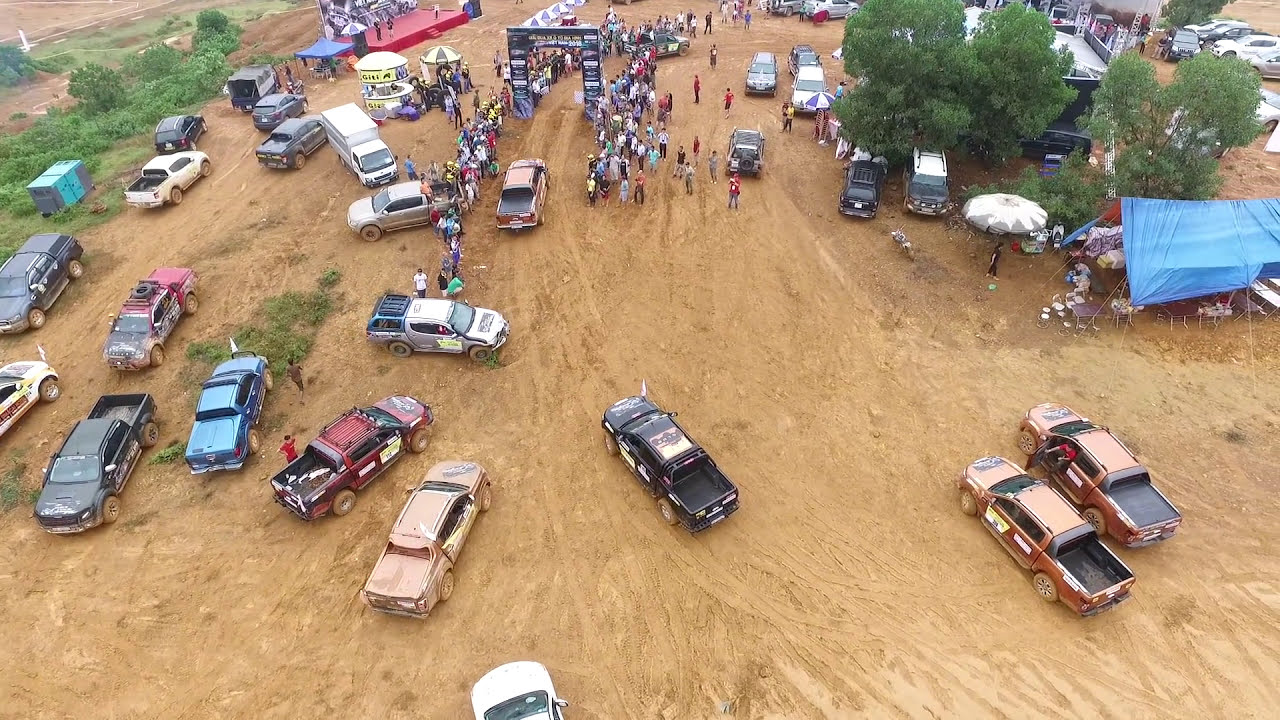This aerial photograph, likely taken from a drone at a height of three to four stories, captures a daytime scene of a large dirt field. The landscape is predominantly light brown, dry dirt with sporadic patches of green grass and a few trees scattered mostly around the outskirts. The focal point is a bustling off-roading event. Trucks and SUVs of various colors, including black, orange, red, and white, are haphazardly parked throughout the field, some bearing the dusty marks of the event. In the upper right corner, a cluster of trees shelters a blue tent and large umbrella, possibly a camping or supply area. Meanwhile, in the upper left corner, a red stage with booths in front of it hosts a gathering of people. Central to the image is a black arch finish line, under which a crowd clad in colorful attire—reds, whites, and blues—eagerly awaits the end of a race. The scene vividly depicts the chaotic energy and communal atmosphere of an off-road rally.